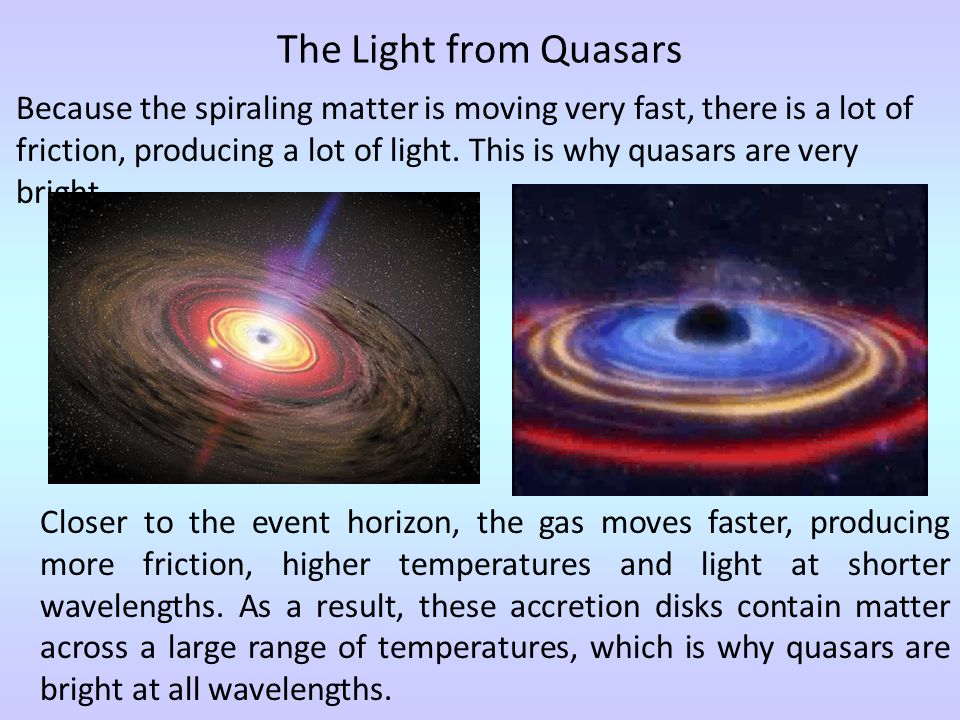The image features a detailed slide about quasars, set against a light purple backdrop that transitions to light blue hues towards the middle. Dominating the slide are two images of spiraling masses, representing quasars, positioned centrally. The left spiral features a bright yellow center, while the right one is illuminated in blue. Both spirals radiate vibrant colors, emphasizing the intense light emitted by quasars. The text on the slide, displayed in dark blue or black font against the light background, describes how the rapidly moving, spiraling matter generates significant friction and, consequently, a lot of light. It explains that closer to the event horizon, the gas speeds up, increasing friction and producing higher temperatures and shorter wavelength light. This results in the accretion disks containing material at varied temperatures, making quasars bright across all wavelengths. Surrounding the main text are stars and hues of yellow, red, blue, black, and white, highlighting the outer space setting of the phenomena.